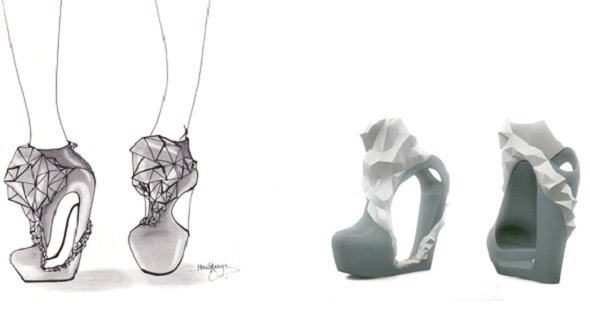The image depicts two sets of fashion shoe representations against a white background. On the left side, there is a detailed pen and ink drawing showcasing a pair of high-heeled shoes worn on legs, stylized in a fashion illustration manner. These shoes are characterized by their exceptionally tall heels that position the feet almost vertically, akin to a ballerina standing en pointe. The shoes feature a blunt nose and a prominent design element on top, possibly a bow or a structured ornament. On the right side, there is a 3D rendering of the same shoes, rendered in shades of gray and white. The 3D model highlights the shoes' dramatic features, including the large hole in the middle and the towering heel, emphasizing their modern, almost sculptural design made of plastic. The absence of legs or feet in the 3D rendering focuses solely on the innovative structure and texture of the shoes, including a white block design element wrapping around the heel, which resembles crumpled paper.